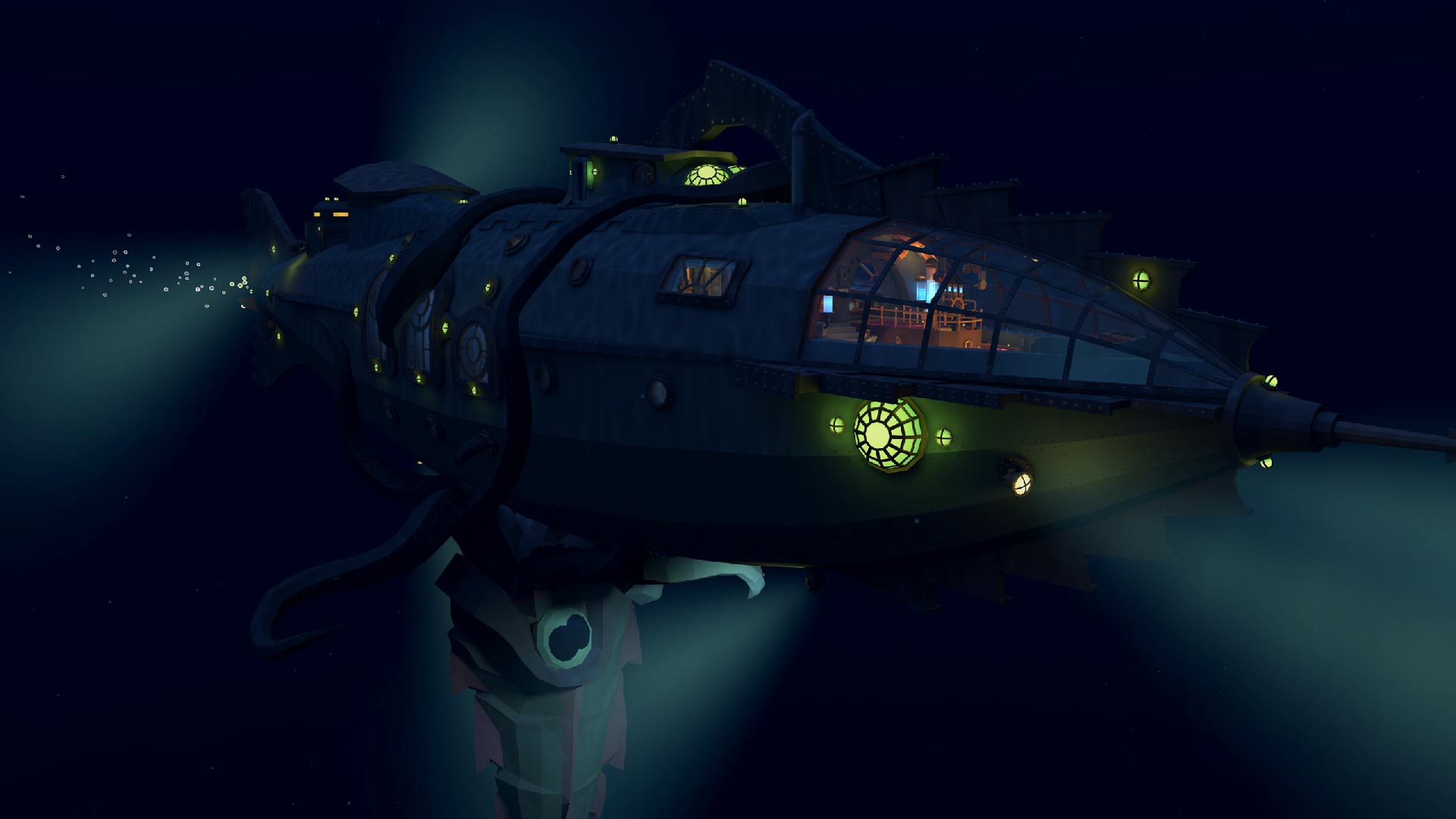This detailed, computer-rendered image captures a mysterious underwater vessel, resembling a wingless plane or submarine, surrounded by a deep, dark blue and black sea. The vessel, illuminated by fluorescent green gears and emitting soft yellowish lights, is depicted with a pointed nose and large cockpit windows through which a single person is visible. Air bubbles trail from the back, while a thick cord anchored to the seafloor extends from underneath. The ominous and dark ambiance is punctuated by misty, bluish-white glows, enhancing the vessel's long, tubular, and enigmatic structure, evoking the scene from a sci-fi movie poster.